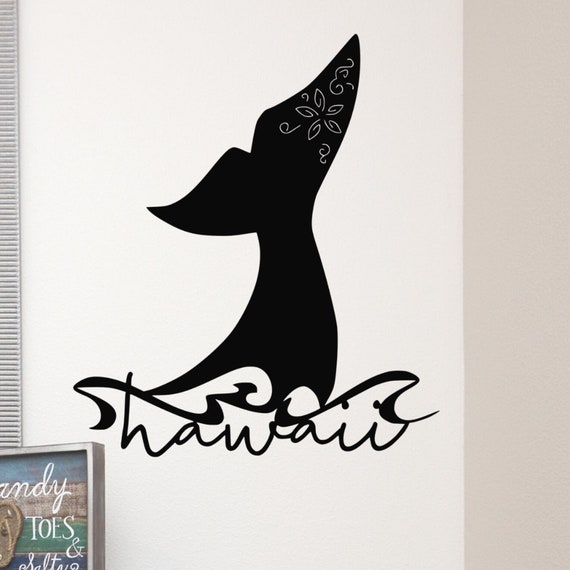The image prominently features a stylized black whale's tail splashing out of the water, rendered in a mostly black and white drawing style. The whale's tail is adorned with an intricate floral pattern on its right fin, characterized by petals radiating towards the center but not connected, accompanied by smaller petals and puffy, cloud-like shapes around them. Sharp, shark-like spikes represent the splashing water, with circular waves emanating to both left and right, emphasizing the dynamic motion. The background consists of a white surface, suggesting it may be a piece of paper or canvas. 

In the bottom left of the image, within a square frame, casual handwritten text spells out "Hawaii" in lowercase letters. A faint brownish object and slightly obscured words, including "Hamdi" and "toes," are also present within this frame, adding more texture to the composition. Additionally, a portion of a gray picture frame with blue and green hues and some white lettering is visible, along with an edge that hints at a wall corner, possibly indicating that the drawing is displayed on a wall in a well-lit room.